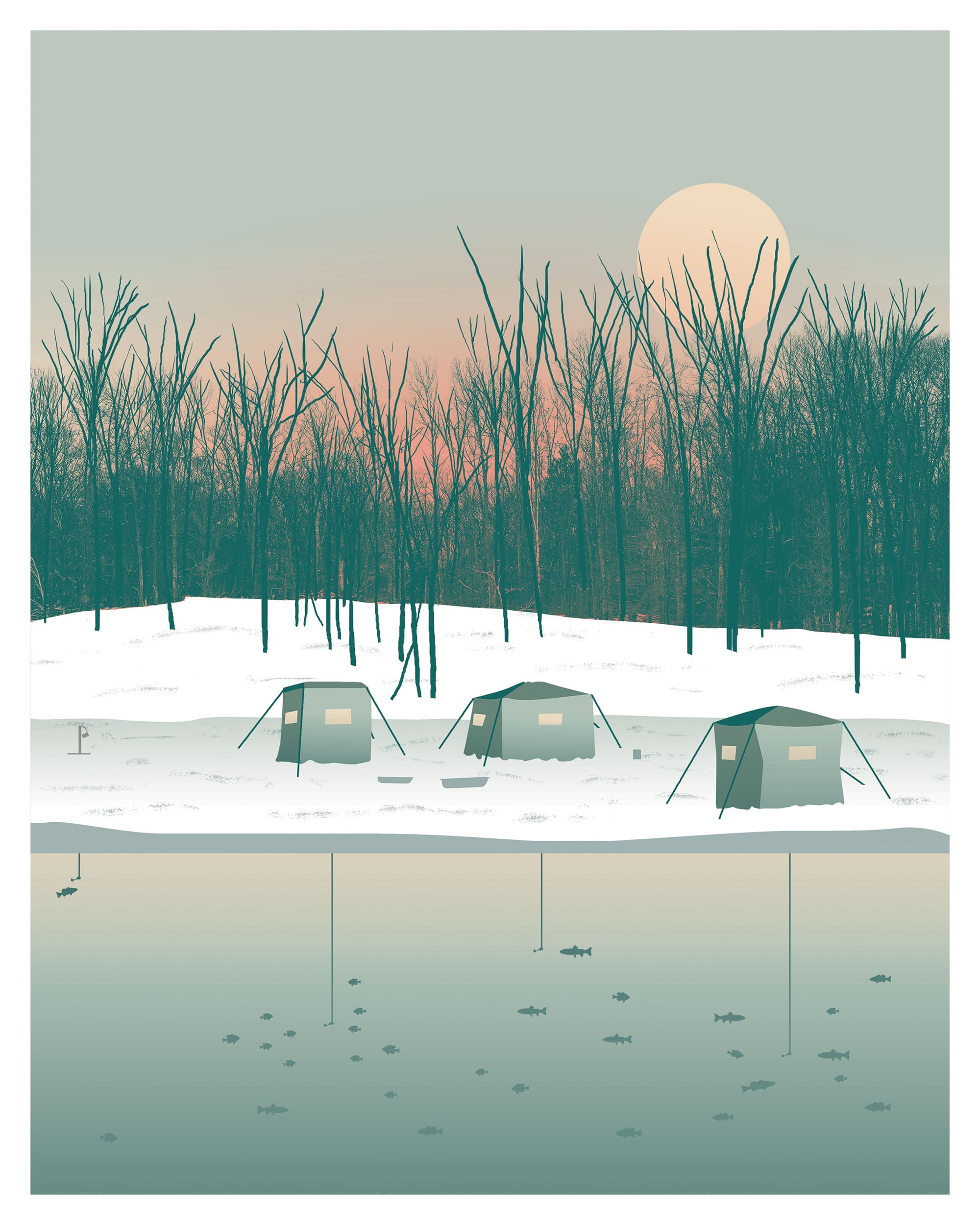This digital artwork, rendered in a vector style, is a detailed vertical illustration of a winter ice-fishing scene. Dominating the composition are three light blue, square-shaped ice fishing tents, each with two visible windows facing inward and to the left. These tents are securely set upon a thick, snow-topped layer of solid ice that forms the surface of a frozen lake. From each of the tents, black fishing lines descend into the blue water below, surrounded by numerous fish swimming near the hooks. On the left side of the lake, there's an additional fishing hole with a line but no accompanying tent, and a single fish appears poised to bite.

Above this lively underwater scene, the sky features a gradient that shifts from an off-blue or light green at the top down to a bright pinkish-orange near the horizon, suggesting the glow of either a setting or rising sun. Offering a calm, wintry backdrop are numerous bare trees, stark and leafless, with a full moon suspended in the top right portion of the image. The white, snow-covered ground and the dark, silhouetted trees convey the chill of the season, tying the entire scene together in a serene yet vibrant display of winter fishing activities.